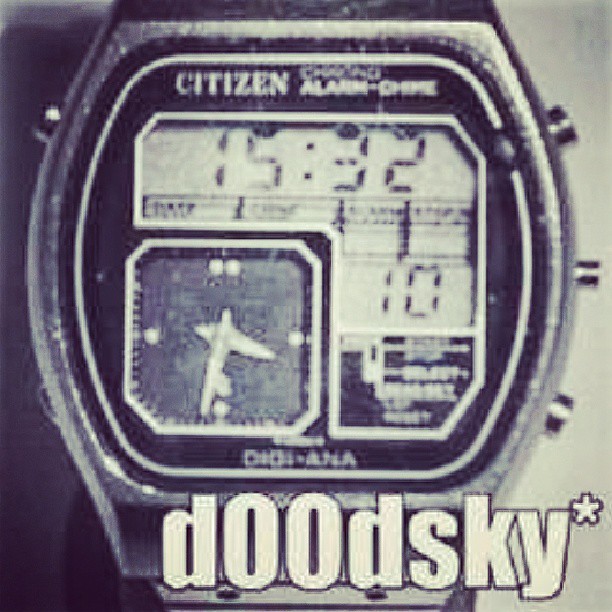This image showcases a close-up view of a Citizen Watch, likely intended as an advertisement. The overall color scheme is monochromatic, dominated by shades of gray, white, and black. The watch itself has a rectangular face with slightly convex sides, bordered by a crisp white outline. 

On the left side of the watch, there is a single adjustment tab, while the right side features three additional tabs for various functions. The brand name "Citizen" is prominently displayed at the top of the watch face, with the word "Alarm" partially visible beneath it, indicating this is an alarm-capable model. 

The digital display shows the time as 15:32, situated immediately below the Citizen branding. Towards the bottom left of the watch face, there's an analog dial set to approximately 3:30. Adjacent to this dial, an additional small LED screen displays the number "10," with some indistinct text beneath it.

At the very bottom of the watch face, the word "Dudeski" is boldly printed, presumably the model name of this particular timepiece. The background of the image is a uniform gray, which further highlights the striking design and details of the watch.